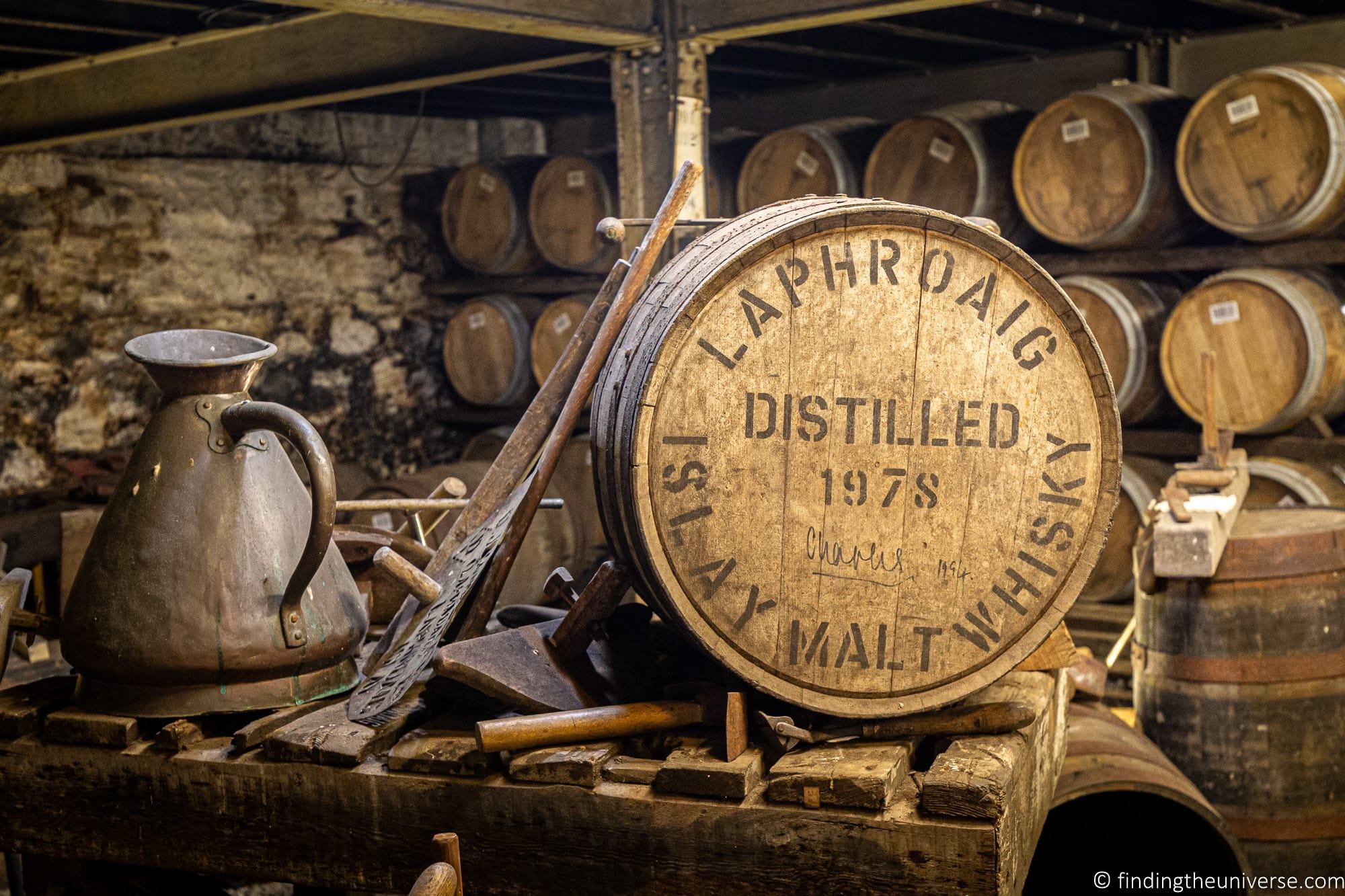The scene depicted is of an old, rustic whiskey distillery or cellar, predominantly bathed in shades of brown, beige, and gold. The walls are constructed from weathered brown bricks, and wooden beams support the partially visible ceiling. In the foreground, resting on a wooden shelf with wide plank separations, is a prominently featured barrel labeled “LAPHROAIG, distilled 1978, Islay malt whiskey.” Nearby lies a tarnished, antique-looking metal pitcher, likely made from old copper. Various other wooden tools and apparatuses, perhaps used in the distillation process, are scattered around. In the background, numerous barrels line the brick walls, stacked on shelves, with some even resting on the ground, all contributing to the historical and provincial ambiance of this whiskey storage space. Additionally, in the far right bottom corner, there is a watermark that reads "findingtheuniverse.com."